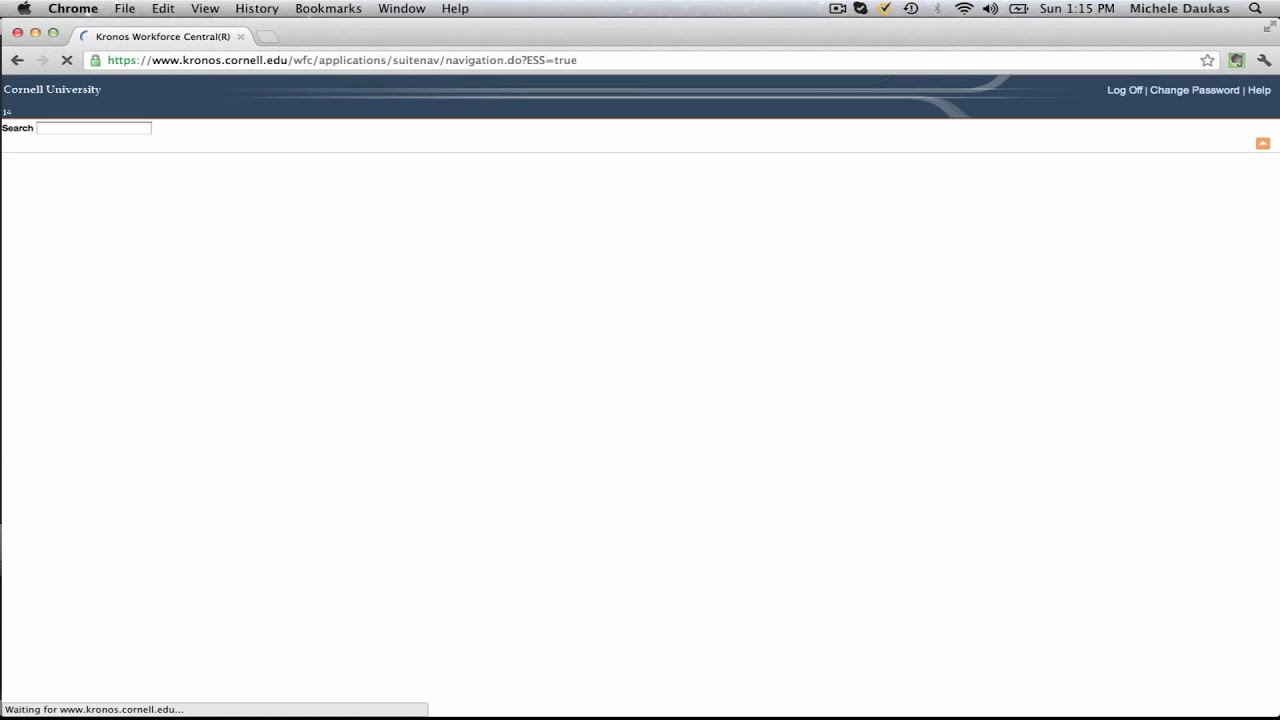Screenshot of a website viewed on a Google Chrome browser on a Mac device, evident from the red, yellow, and green close-minimize buttons at the top left. The browser tab reads "Kronos Workforce Central" and the URL is www.kronos.cornell.edu, indicating a Cornell University site. The top left of the webpage displays "Cornell University" with a dark blue header featuring two overlapping screen-like effects. Below this, there's a section that reads "One ~" suggesting a possible title or section header. At the top right, options for "Log Off," "Change Password," and "Help" indicate the user is logged in. Beneath the header, there's a search bar without any input, hinting that the page may not have fully loaded the content. The incomplete loading suggests a potential error on the site.